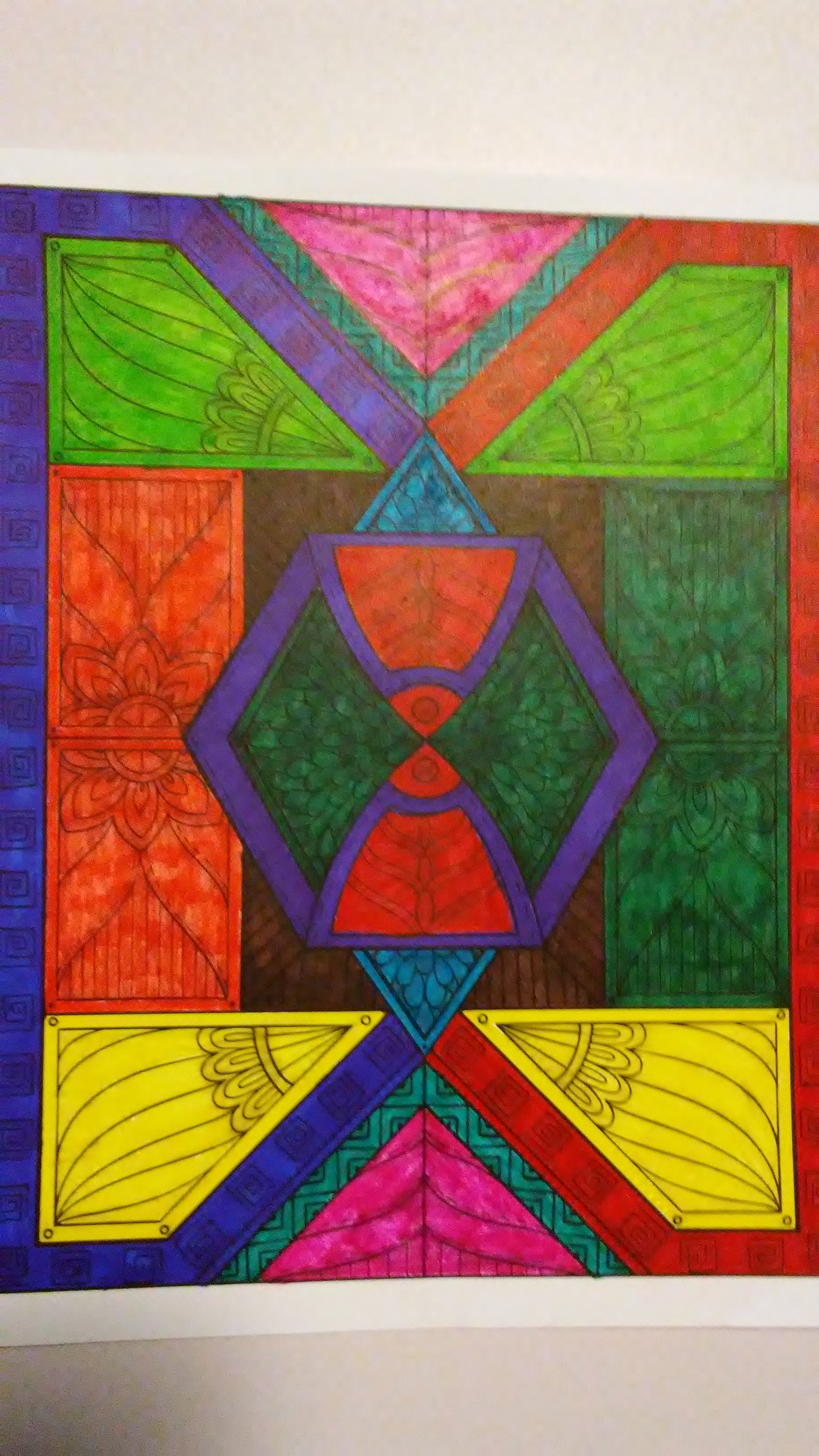This captivating piece of artwork, meticulously crafted on white paper, showcases a rich tapestry of geometric designs brought to life with vibrant colors. At the heart of the composition lies a central hexagon, its bold shape commanding attention and forming the focal point of the artwork. Radiating from this central hexagon are various geometric shapes, including a diamond positioned directly below it. Enhancing the symmetry, two triangles extend from the top and bottom sides of the hexagon, creating a balanced yet dynamic visual.

Encircling the entire artwork is a distinctive border that further accentuates the vibrant central patterns. The left border is a striking dark blue, adorned with intricate black swirls that add depth and intrigue. In contrast, the right border features a rich dark red, also embellished with black swirls, creating a harmonious yet contrasting frame.

Flanking the hexagon on either side are pairs of vertically aligned rectangles. On the left, the rectangles are painted a deep red and are intricately decorated with a delicate floral design, adding an element of natural elegance. On the right, the rectangles are a lush green, similarly adorned with floral motifs, creating a visually pleasing symmetry and balance within the piece.

This artwork is a masterful blend of geometric precision and vibrant creativity, making it a visually captivating and richly detailed composition.